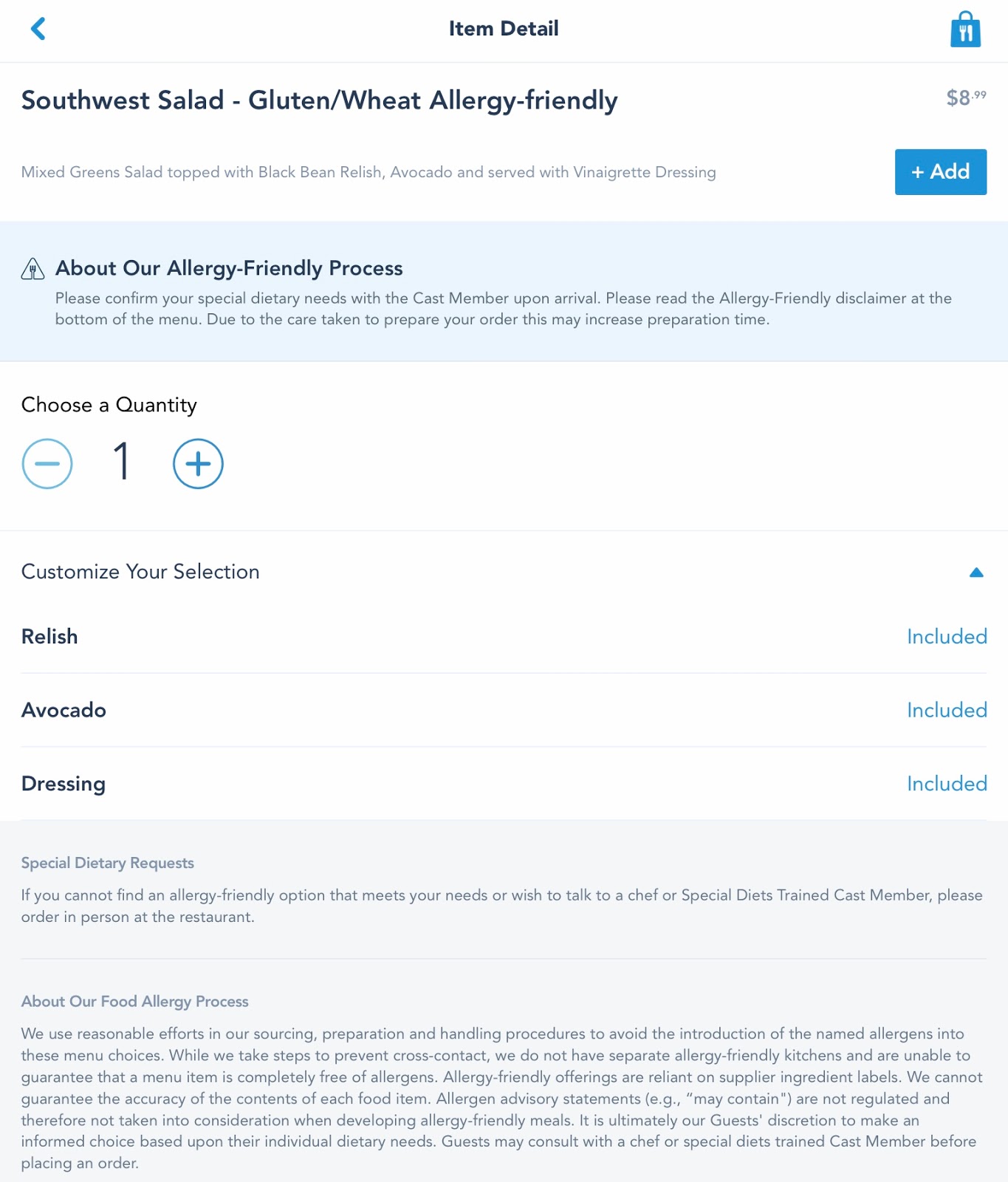**Detailed Caption:**

The image showcases a primarily white background with several notable elements, starting with a blue arrow pointing to the left-hand side. On the right side, a blue icon resembling a shopping bag with a white knife and fork indicates a food purchase option. A thin gray line separates sections of the content.

In dark blue text, the title reads "Southwest Salad - Gluten/Wheat/Algae-Friendly." Below this, in gray, is the price: "$8.99." A detailed description follows in smaller gray text: "Mixed Green Salad Topped with Black Bean Relish, Avocado, Served with Vinaigrette Dressing."

Further down, a blue rectangular button with white text prompts users to "+ Add." A light blue background contains information about the allergy-friendly process, stating: "About our Allergy-Friendly Process. Please confirm your special dietary needs with the cast member upon your arrival. Please read the Allergy-Friendly Disclaimer at the bottom of the menu. Due to the care taken to prepare this order, this may increase preparation time."

In black text, guidance for choosing quantity is provided: "Choose a Quantity" with a default of "1" and two circles featuring minus and plus signs for adjustment. Another section encourages customization: "Customize Your Selection" followed by "Relish," "Avocado," and "Dressing" with each ingredient having a blue "Include" button next to it.

At the bottom in gray text, there is an advisory: "Special Dietary Requests. If you cannot find an Allergy-Friendly option that meets your needs, or wish to talk to Chef or Special Dietary Cast Member, please order in person at the restaurant."